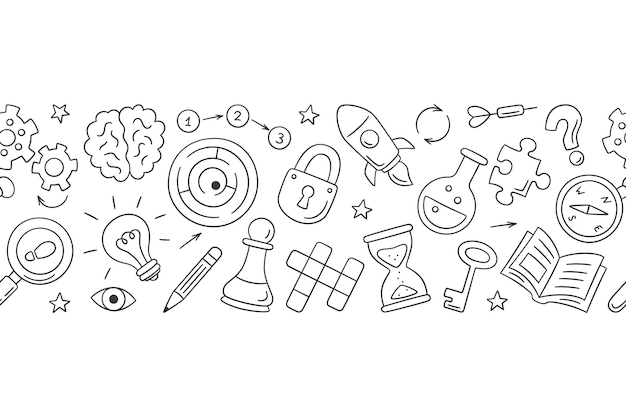This black and white image, set within a rectangular frame, is a collection of intricate black sketches spread across the page in no particular order, resembling a page from a coloring book. The minimalist drawings feature a mix of everyday items and symbols: gears both on the top left and scattered throughout, representing cogs inside a clock or a mechanism; stars sprinkled across the entire image; and a jigsaw puzzle piece. There is also a sharp-edged dart akin to a syringe, multiple arrows including a circular cycle of arrows, and an eye. Notably, a compass tilted with its 'N' facing the upper left corner, a key, and an hourglass are present. A blank crossword puzzle and stars appear at various points, as well as a chess pawn and a light bulb emitting rays to indicate illumination. The bottom section includes a book depicted with lines to suggest text, a pencil, a beaker with bubbling contents, and a magnifying glass with a footprint inside. Additional elements such as a brain, question marks, rockets, and a segment that looks like a maze complete the eclectic assortment of doodles.